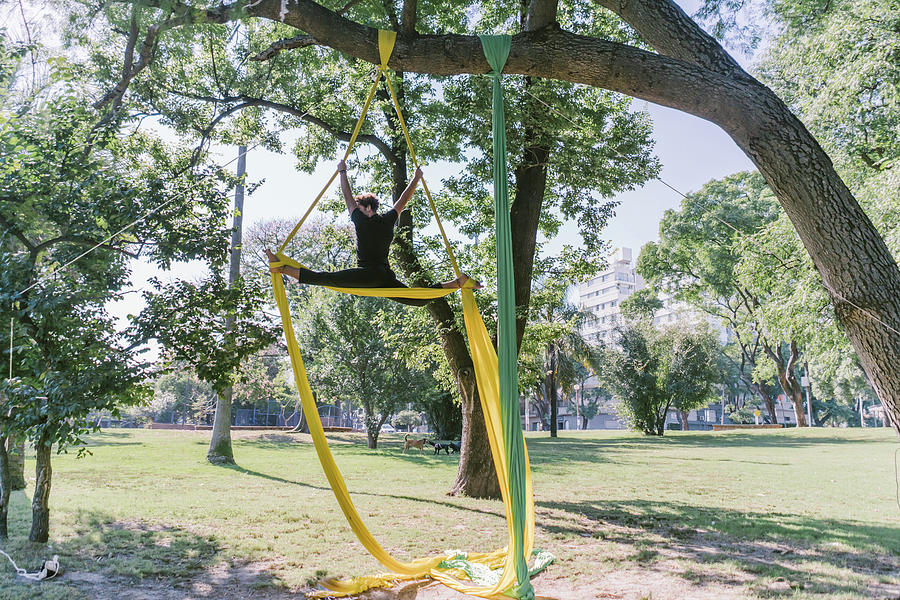In this wide shot of a downtown urban park, vibrant with sprawling green grass and many diverse trees, a striking scene unfolds beneath a tree with gracefully curving branches. Two long pieces of fabric, one yellow and one green, hang suspended from the tree's branches. The yellow fabric cradles a man with short wavy hair, donned in black clothing. He is performing an acrobatic display, with his arms outstretched in a Y shape, gripping the top of the fabric, and his legs in a full split. His pose resembles that of a ballerina, showcasing his athleticism and grace amidst the serene park setting. In the far distance, tall white high-rise buildings frame the skyline, highlighting the park's urban location. Additional details include the green fabric hanging unused beside him, and two small dogs barely visible, wandering in the far reaches of the park.